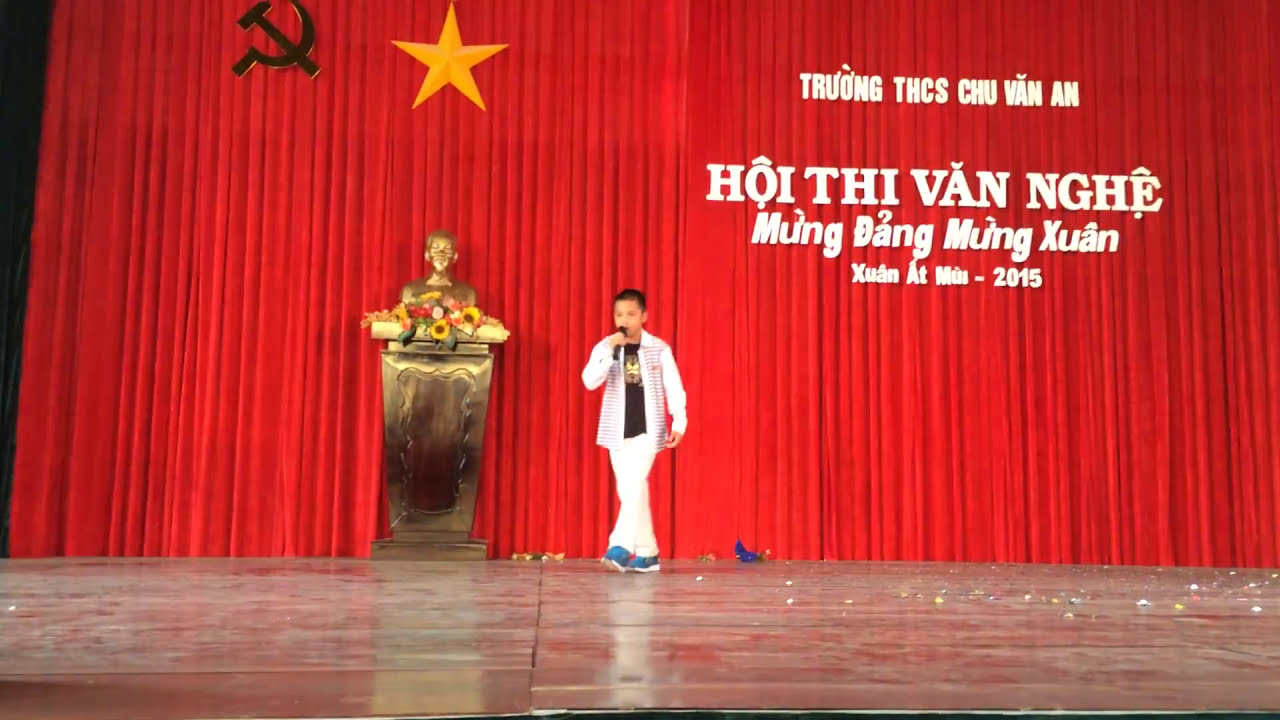A young man with dark hair, dressed in an open white jacket over a black shirt and white pants, is standing on a stage and speaking into a microphone held in his right hand. He wears blue sneakers. The backdrop is a heavy red curtain adorned with communist symbols—a hammer and sickle crossed together and a yellow star—on both the left and right sides. To the left of the young man, there is a golden podium adorned with a gold bust surrounded by flowers. The red curtain behind him features Vietnamese text, including sequences that read "Truong THCS Chu Van An," "Hoi THI Van NGHE," "Mung Bang Mung Xuan," and "Xuan am M-2015."